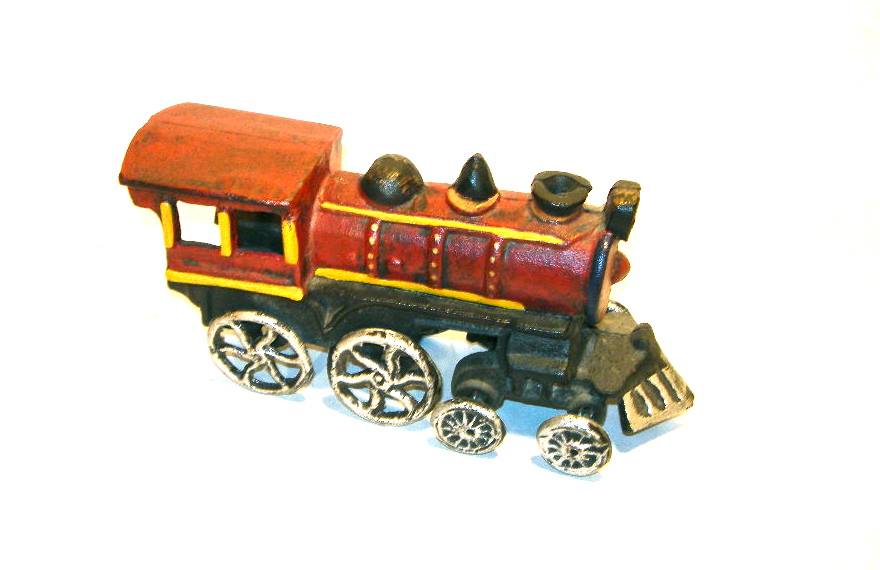Here is a detailed caption for the image:

"This intricate drawing depicts an old-fashioned toy train, facing towards the right. The train is predominantly red and features a classic design, complete with a cow catcher at the front. The undercarriage includes two small white wheels at the front and two larger wheels towards the back. On the left-hand side of the image, there is a cage-like cabin where the train operator would sit. In front of this cabin, the train's body is cylindrical, adorned with three distinct dark gray extensions on the top. The first extension is semicircular, the second has a triangular shape, and the third is a flat-topped, gray rectangle. These extensions are not very tall, complementing the overall compact and detailed aesthetic of the toy train."